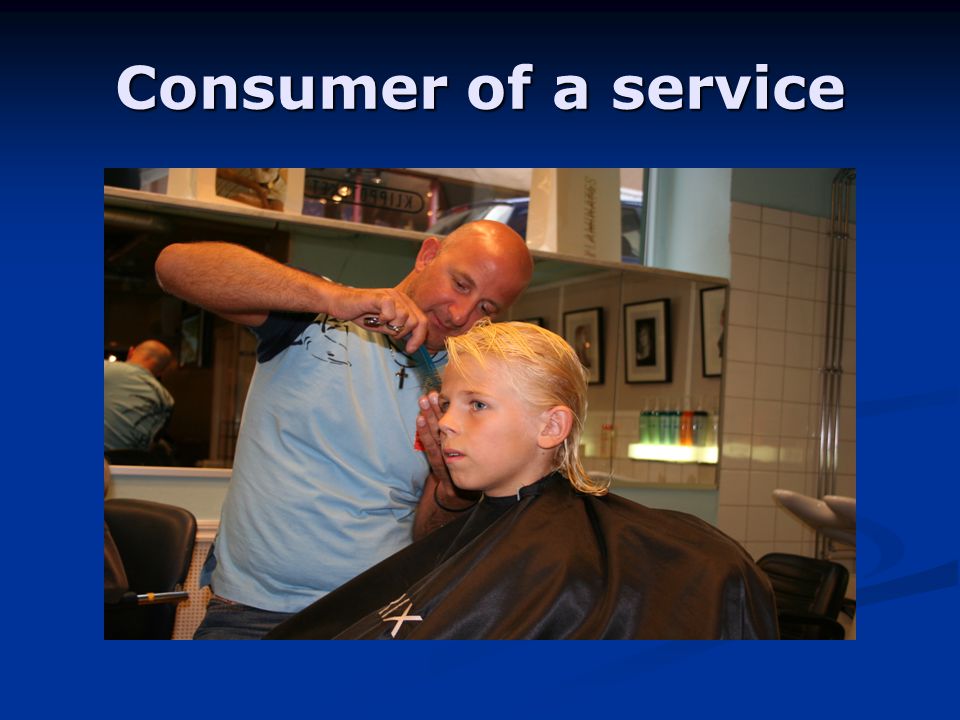The image is a square with a blue border that reads "Consumer of a Service" in white lettering. It depicts a scene in a salon, where a bald man in a light blue shirt, adorned with a cross necklace, is giving a haircut to a young boy with blonde hair. The boy, who looks subtly expressive, is seated in a barber's chair wearing a black cape to catch the hair, which has white letters on the front. Their setting includes a wide mirror behind them, reflecting shampoo bottles and photos of different hairstyles, as well as a window above the tiled wall, through which a car can be seen.